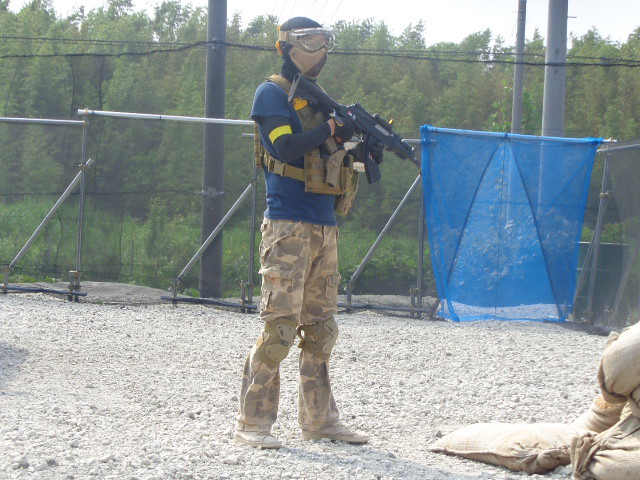The image depicts an individual at what appears to be an airsoft field or possibly a military training site. The person is wearing a blue long-sleeve shirt beneath a bulletproof vest and camouflage pants, accompanied by white shoes. Their face is mostly obscured by a mask with a glass shield covering their eyes, rendering their gender indistinguishable. The individual is holding what looks like an automatic airsoft gun, potentially an AK-47 style replica.

The scene is set during the day under a light gray sky, with a distant backdrop featuring a dense line of green pine trees. In the immediate background, there is a woven fence supported by multiple tall metal poles, from which a black netting or blue mesh is draped, likely serving as a barrier. The ground is covered in gravel, and a pile of burlap sandbags is visible at the far right, adding to the setting's realistic or militarized ambiance.